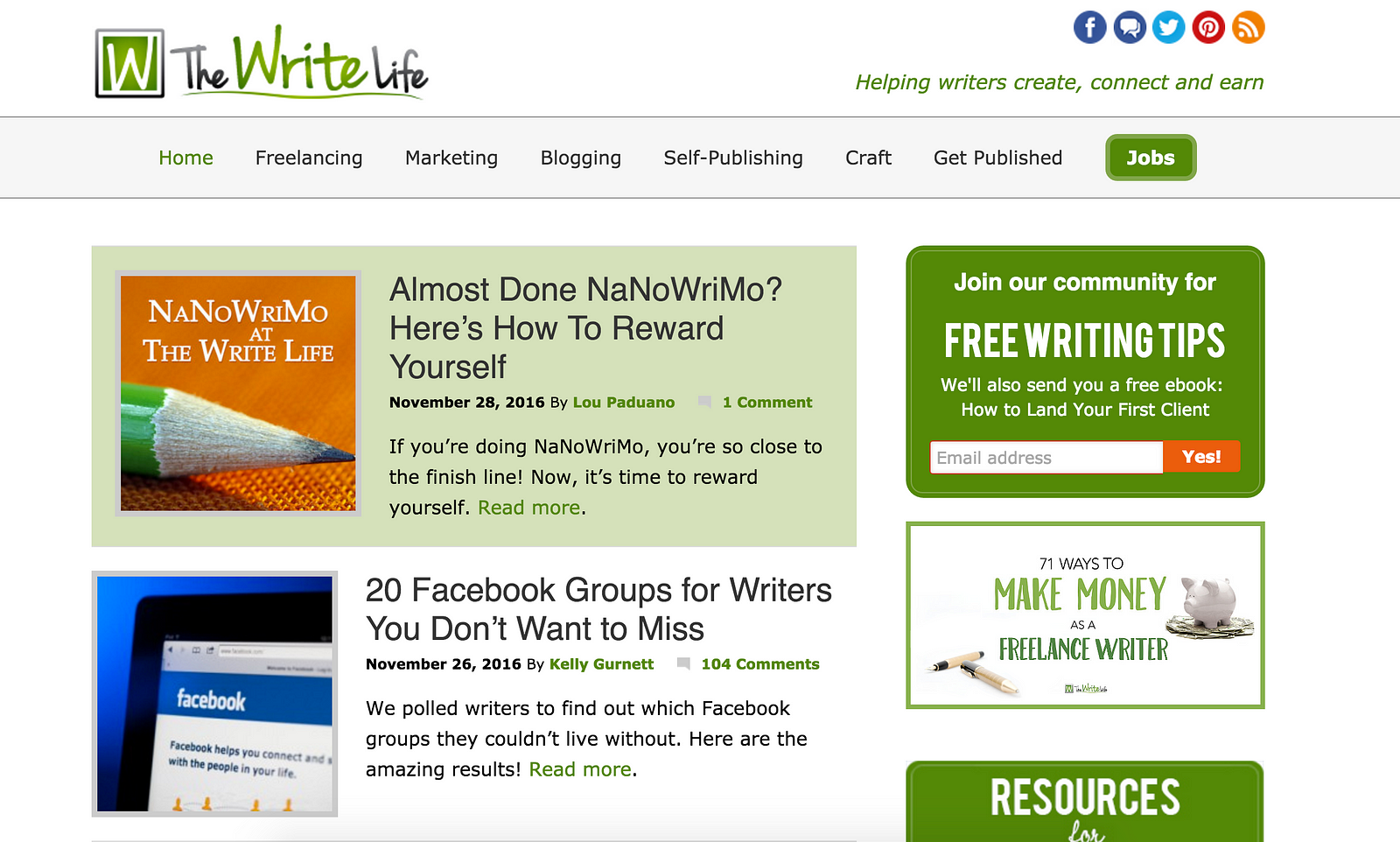This image is a screenshot from a website titled "The Write Life." In the upper left-hand corner, there's a logo featuring a green box with a black outline and a white letter "W" inside the green area. Next to the logo, the website name "The Write Life" is displayed, with "Write" written in a handwritten style and colored green.

To the right of the logo are various social media icons for the website’s contacts, including Facebook, Twitter, RSS feed, and Pinterest. Below this section is a navigation bar with clickable text links directing to different areas of the website. The homepage is currently highlighted, but other links include Freelancing, Marketing, Blogging, Self-Publishing, Craft, Get Published, and a distinctive green button labeled "Jobs."

Beneath the navigation bar, there's a prominent link to an article featured in a long rectangular box. The box contains an image of a pencil tip and the phrase "NaNoWriMo at The Write Life." Accompanying the image is the title of the article: "Almost Done with NaNoWriMo? Here's How to Reward Yourself." The article is dated November 28, 2016, authored by Lou Padowano, and has one comment. Users can click on this link to read the full article. Below this, another article link is partially visible, indicating additional content follows.